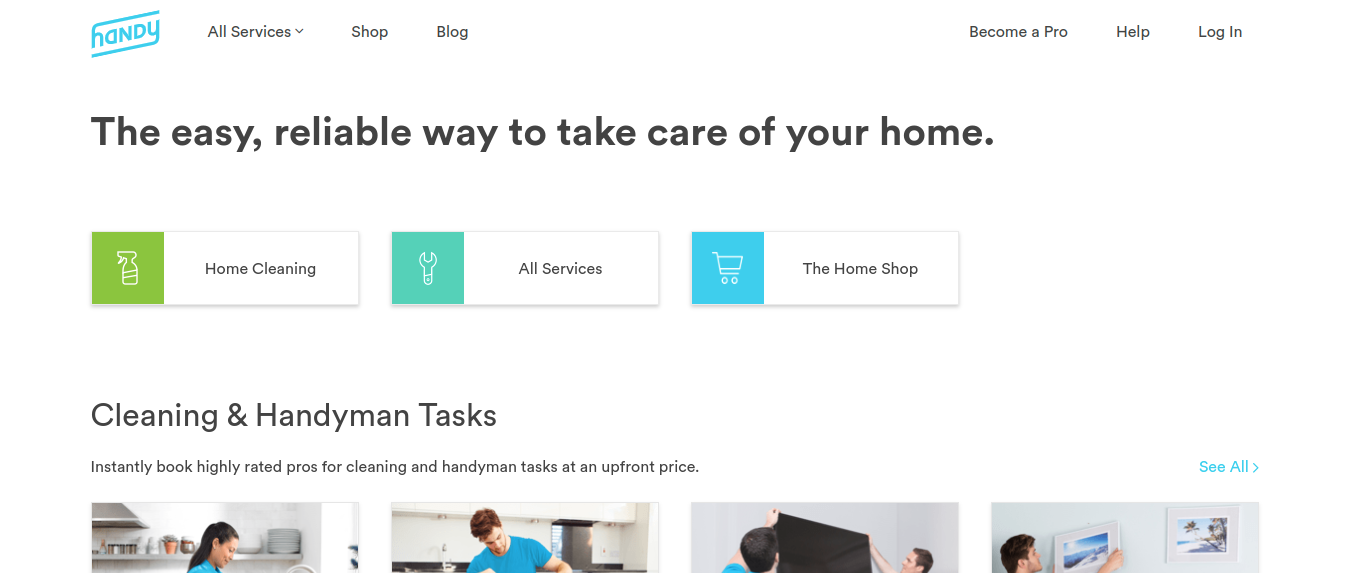This screenshot captures the top section of a webpage with a clean, solid white background. In the top left corner, "Handy" is prominently displayed in light blue text, with an understated line running beneath the 'H' and 'Y', forming a subtle rectangular highlight. 

At the top-center of the page, a navigation menu includes options for "All Services" (indicated by a downward-pointing arrow for a dropdown menu), "Shop," and "Blog." On the right side, three horizontal boxes offer additional options: "Become a Pro," "Help," and "Log In."

Directly below this main navigation, three distinct horizontal boxes provide quick access to specific services. The first box features a pea green spray bottle icon against a white background, labeled "Home Cleaning" in black text. The second box, in a teal hue, includes a white wrench icon and the label "All Services." The third box is light blue, showcasing a white shopping cart icon and the words "The Home Shop."

Further down, the page offers a brief description of available services under the heading "Cleaning and Handyman Tasks," highlighting the range of tasks users can request. Finally, a series of four images along the bottom showcase individuals performing various tasks; however, each image is truncated roughly one quarter from the top.